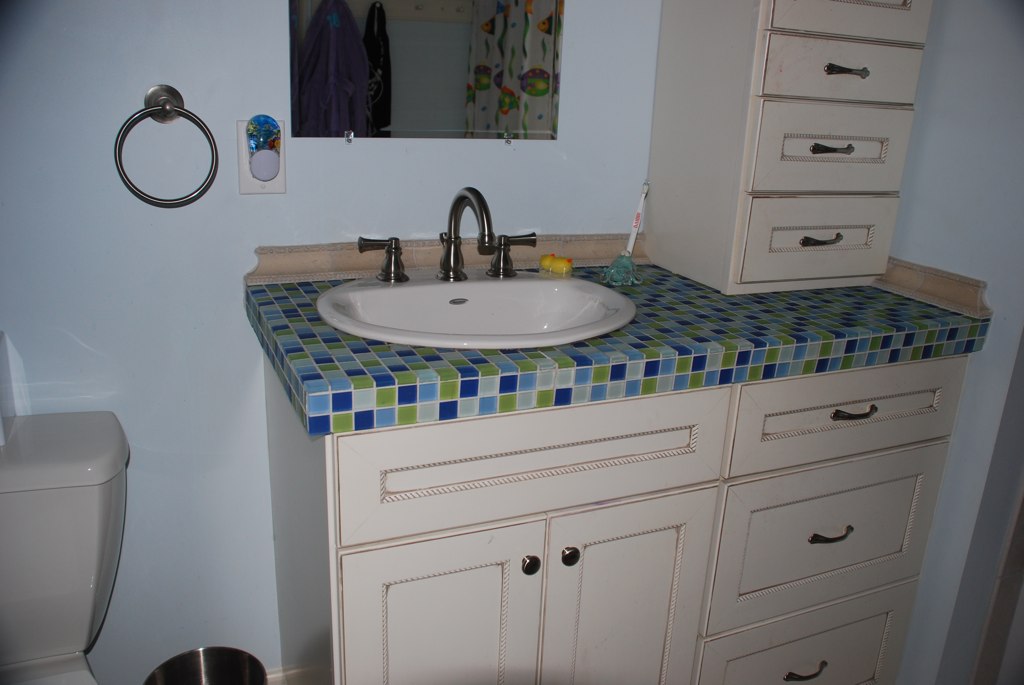This image depicts a bathroom with several distinctive features. Central to the composition is a bathroom mirror mounted on the upper middle section of the wall. The mirror reflects the opposite side of the bathroom, revealing a light brown shelf attached to the wall with several hooks. On these hooks hang two items: a purplish bathrobe and a black sweater-like garment. The bathroom walls are painted a light blue, adding a calming atmosphere to the space.

To the right, there is a white shower curtain adorned with bird designs, giving the area a whimsical touch. Below the mirror, situated in the middle of the image, is a white sink fitted with silver knobs and faucets. The sink rests on a countertop with a multicolored checkered pattern incorporating shades of green, blue, and white, adding a vibrant yet cohesive look.

Below the countertop are light tan shelves, which are organized into distinct sections. On the bottom right, three horizontal shelves are stacked vertically, while two additional shelves are located on the bottom left. More storage is visible at the top right corner of the counter, featuring horizontally oriented rectangular shelves positioned vertically. The bathroom's blend of functional storage, soft color palette, and decorative elements create a warm, inviting space.